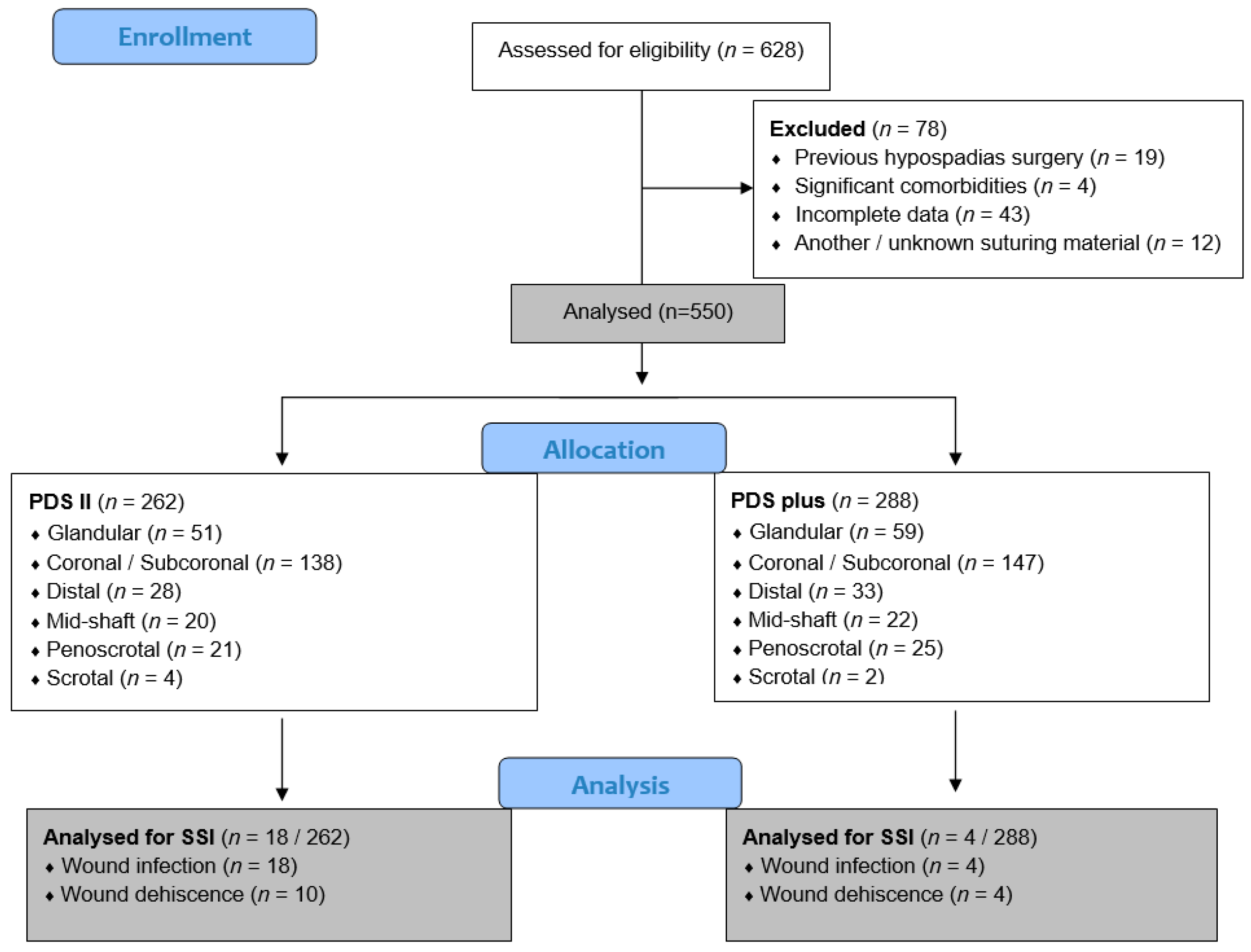The image features an extensive flowchart, likely part of a research paper, academic journal, or a presentation slide, detailing a medical process. The chart begins with a large central box at the top labeled "Assessed for Eligibility (N = 628)," which branches out into various sections. On the left side of this starting point, a rounded blue box labeled "Enrollment" initiates the diagram's flow. 

To the right of the "Assessed for Eligibility" box, another section labeled "Excluded" notes the number of subjects who were not included in the study. Below the initial box, a box labeled "Analyzed" (possibly around N = 500 or 550 subjects) splits into two distinct paths, each diverging left and right into subcategories. These subcategories fall under a section titled "Allocation," also marked with a rounded blue box. Each of these paths then leads down to additional sections under the "Analysis" category.

The boxes in the "Analysis" section at the bottom are slightly grayed out, contrasting with the white boxes above. These details, along with arrows guiding the flow from one step to another and complex medical terminology, suggest the chart outlines a detailed and structured medical protocol or policy.